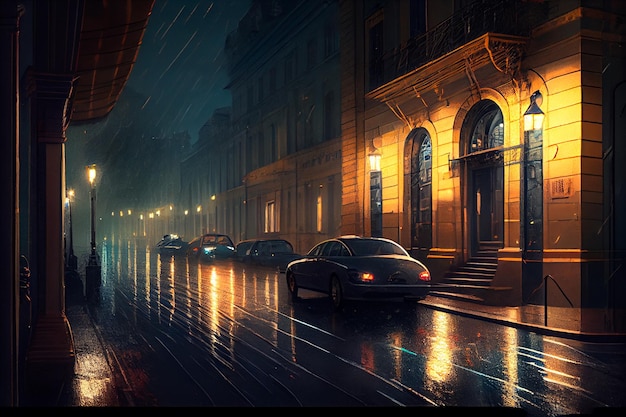This image, which may be a painting or computer-generated, depicts a rainy night on a city street, possibly European. The scene, seen from a high vantage point, features rain streaking diagonally through the dark sky, creating a moody atmosphere. The street below is flanked by tall, multi-story buildings, their façades obscured in darkness except for one notable stone building brightly illuminated by fluorescent lights. On both sides of the road, street lights cast a subdued glow, and reflections of rain glisten on the wet concrete. Cars, varying in style from futuristic to vintage, are parked along the sides of the street; three are visible in the distance, with one parked closer in the foreground. One building, distinct with its yellow brick and two large black arched doors, exudes a warm yellow light, contributing to the scene's mysterious allure. The overall effect is evocative and detailed, with a striking juxtaposition of light and shadow across the urban landscape.